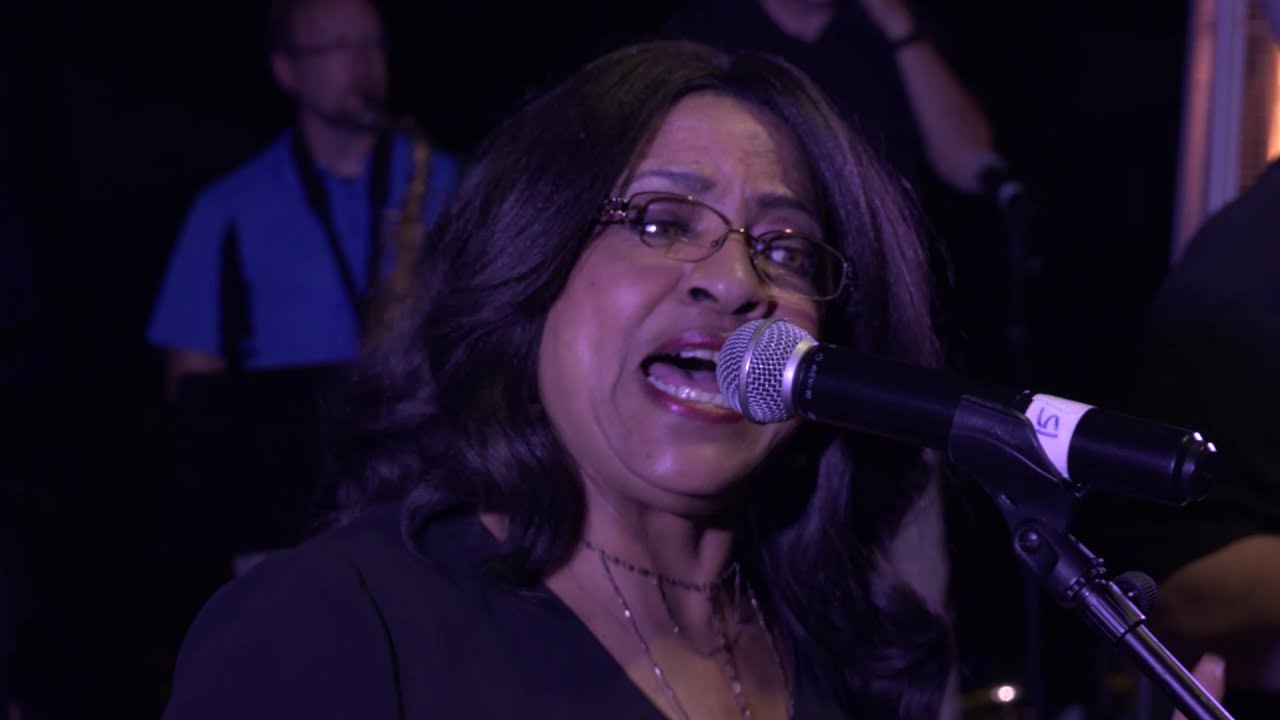In this captivating photograph taken in a dimly lit setting, a woman of African descent, possibly in her 50s or 60s, sings intently into a black and silver microphone adorned with a white sticker featuring the number 15 in blue. The microphone is mounted on a black stand and is positioned close to her face. Her dark, shoulder-length curled hair frames her face, and she wears eyeglasses and brown lipstick. Dressed in a black v-neck blouse and a silver chain necklace, her concentration is evident as she focuses on delivering her song, seemingly looking past the camera towards an unseen audience.

To her left, there are several background figures. One man, wearing a blue shirt and glasses, has a guitar strap around his shoulder and a black rope around his neck. Another man, dressed in a black short sleeve shirt, is visible by his arm, and a third figure appears to be raising his arm towards his face. The scene suggests a collaborative performance, possibly on a late-night talk show or in an informal choir setting.